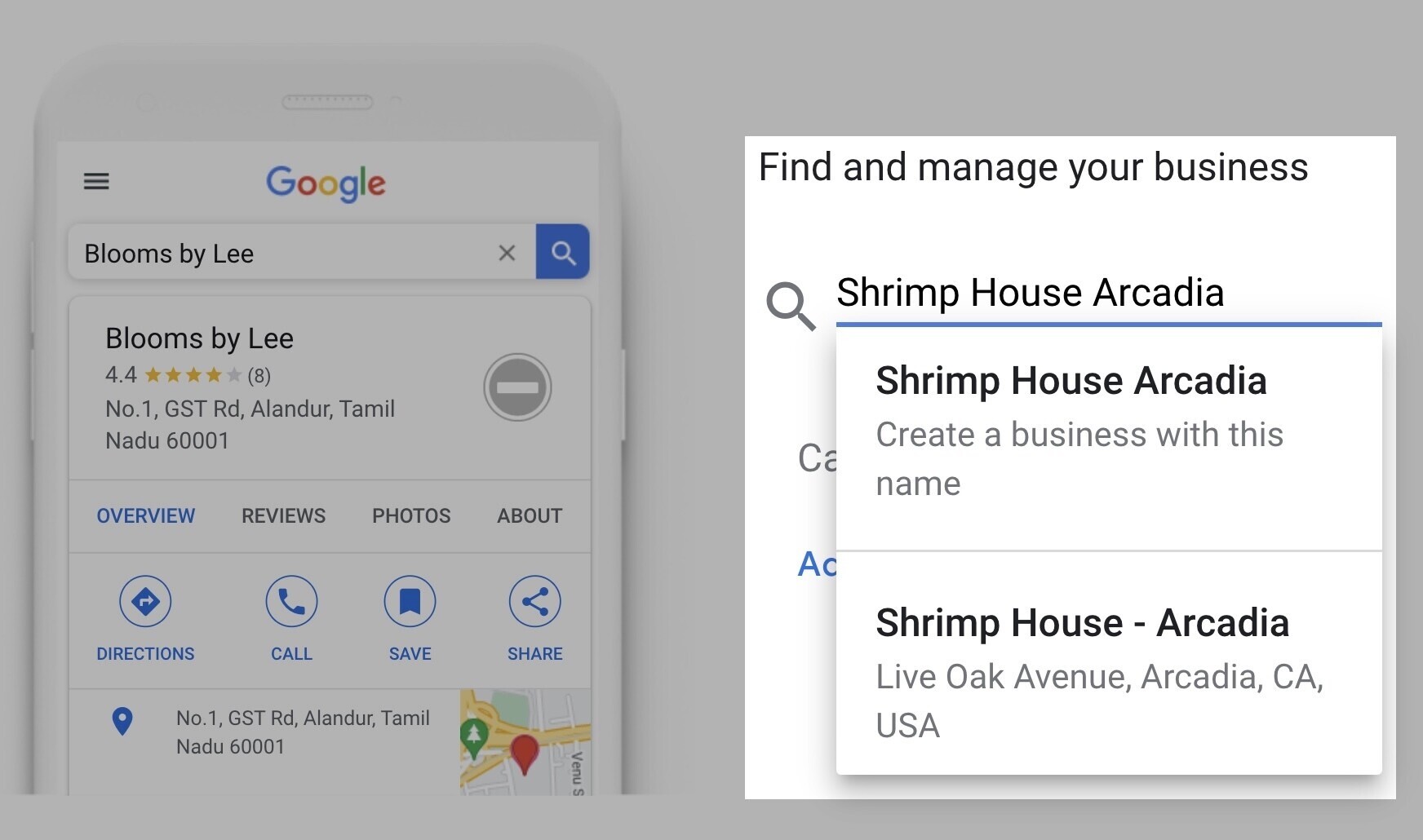The image shows a screenshot of a mobile phone displaying the Google interface. At the top left corner, there is a hamburger menu icon. Beneath that, a text box displays "Blooms by Lee" with a blue button of the same name. The interface includes various tabs labeled "Overview," "Reviews," "Photos," and "About." Below these tabs, there are buttons for "Directions," "Call," "Save," and "Share."

On the right side of the screen, a section reads "Find and Manage Your Business" in full opacity. In the search input box, the business name "Shrimp House Arcadia" is entered. An overlay appears, showing suggested auto-populated categories, including "Shrimp House Arcadia," an option to "Create a business with this name," and another listing for "Shrimp House Arcadia" located at "Live Oak Avenue, Arcadia, California, USA." The interface combines business information and management features in a user-friendly layout.